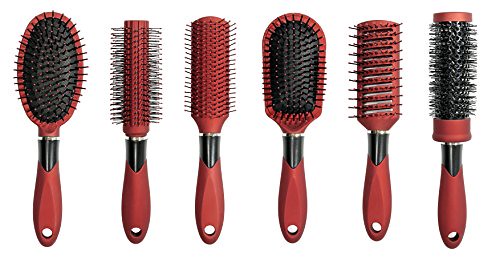This photograph features six distinct hairbrushes neatly aligned side by side against a white background. Each brush shares a common design language with brownish-red handles accented by a black section and a hole at the bottom of the handle. Starting from the left, the first brush is an oval-shaped detangling brush with dense black bristles. Next is a round brush with black bristles encircling the cylindrical body, ideal for curling hair while using a hair dryer. The third brush is a smaller, rectangular brush with fewer black bristles, suitable for finer styling. Following that is a paddle brush with a square shape that flares slightly at the top, rounded edges, and black bristles, designed for regular brushing. The fifth brush is an open-vented rectangular brush, featuring lines cut through the body to allow airflow, equipped with black bristles for quicker drying. The final brush on the right is another cylindrical round brush, similar to the second one, with thick black bristles for curling hair during blow-drying. The unified color scheme and design details create a cohesive yet varied toolkit for different hair styling needs.